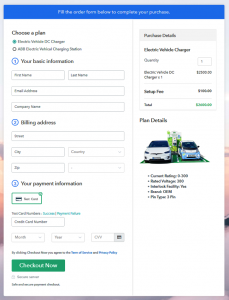The image is a small rectangular vertical format. At the top, there is a narrow horizontal section in bright blue with an indiscernible white font due to its small size. Below this, the page layout is divided into two sections: the left section occupying two-thirds of the width and the right section taking up the remaining one-third.

In the left section, the title "Choose a Plan" is prominently displayed in dark font, followed by two options listed beneath it. The first option is selected, indicated by a filled green dot. Below this, the words "Your Basic" are visible, but the following text is illegible. The section then features fields labeled "First Name," "Last Name," "Email Address," and "Company Name" for user information entry. Further down, there is a space designated for payment information. At the bottom of this section is a horizontal green box with the text "Check Out Now" in white font.

The right section, occupying the final third of the width, is likely labeled "Package Deals" in black font. It lists several items, which are too small to discern clearly. However, the phrase "Plan Details" is visible, accompanied by an animated image of two cars facing forward, with some text beneath this image, also too small to read clearly.